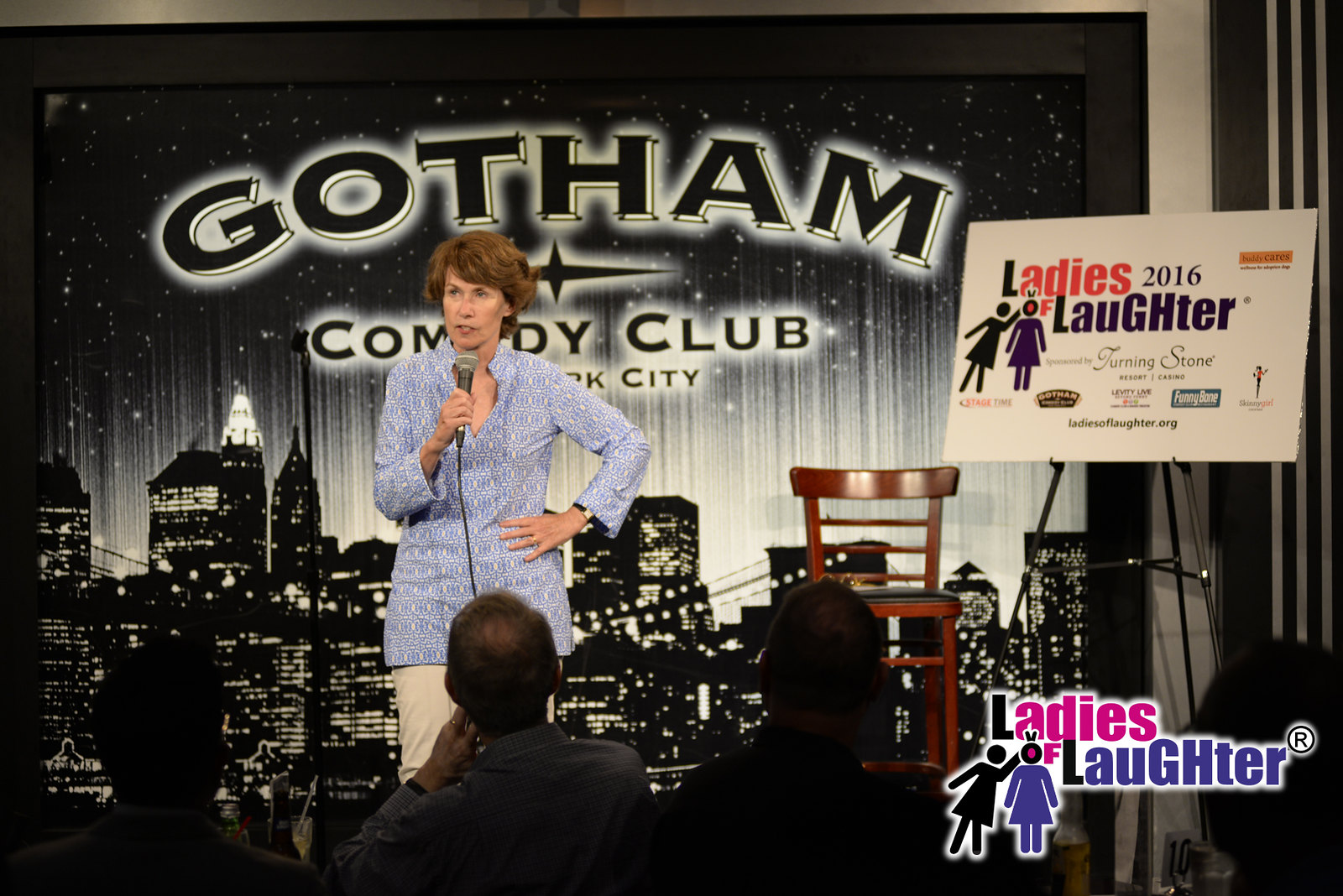The image showcases an older woman with short red hair standing on stage at the Gotham Comedy Club in New York City. She is holding a microphone up to her mouth and is attired in khaki pants and a long-sleeve, tunic-like collared shirt with a blue and white print. The backdrop behind her features a black and white illustration of a New York City skyline, illuminated with lit-up windows and labeled with the text "Gotham Comedy Club New York City" in a serif font. To the right side of the image is a large white sign that reads "Ladies of Laughter 2016," along with additional details like "Turning Stone Resort Casino," Gotham Comedy Club," and "Ladies of Laughter .org," accompanied by silhouettes of two women. The bottom right corner also sports a smaller "Ladies of Laughter" logo with distinctive pink and purple lettering. The setting is a comedy club, and partially visible at the bottom of the image is the engrossed audience focusing on the woman.